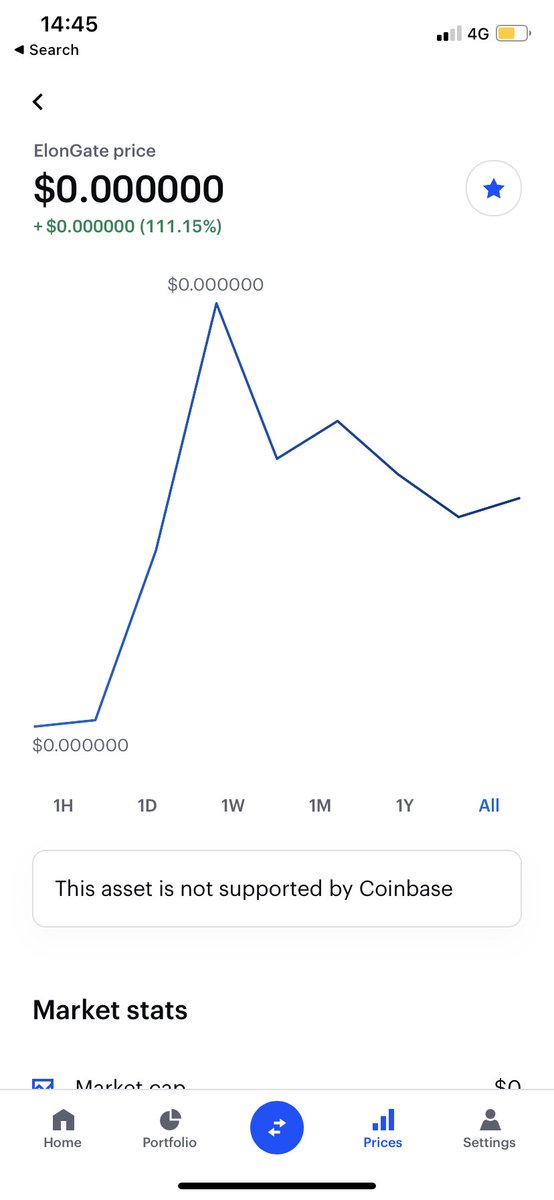This detailed caption describes the given image as follows:

---

The image is a screenshot from a cryptocurrency app, most likely viewed on an iPhone, characterized by its white background. At the top, the status bar indicates the time as 14:45, with the device having two bars of service on a 4G network and approximately 50% battery life remaining. Below the status bar, the application displays the title "Elon Gate Price," referencing a play on words involving Elon Musk and the term "gate."

The price displayed for Elon Gate is 0.000000. Beneath the price, there is a bar graph showing the cryptocurrency's performance over various timeframes: one hour, one day, one week, one month, and one year. Although the graph shows a sharp increase within the one-week mark with a blue line spiking to the top, the values remain 0.000000 across the board.

At the bottom, a message indicates that "This asset is not supported by Coinbase," suggesting that users cannot trade this particular cryptocurrency on the Coinbase platform.